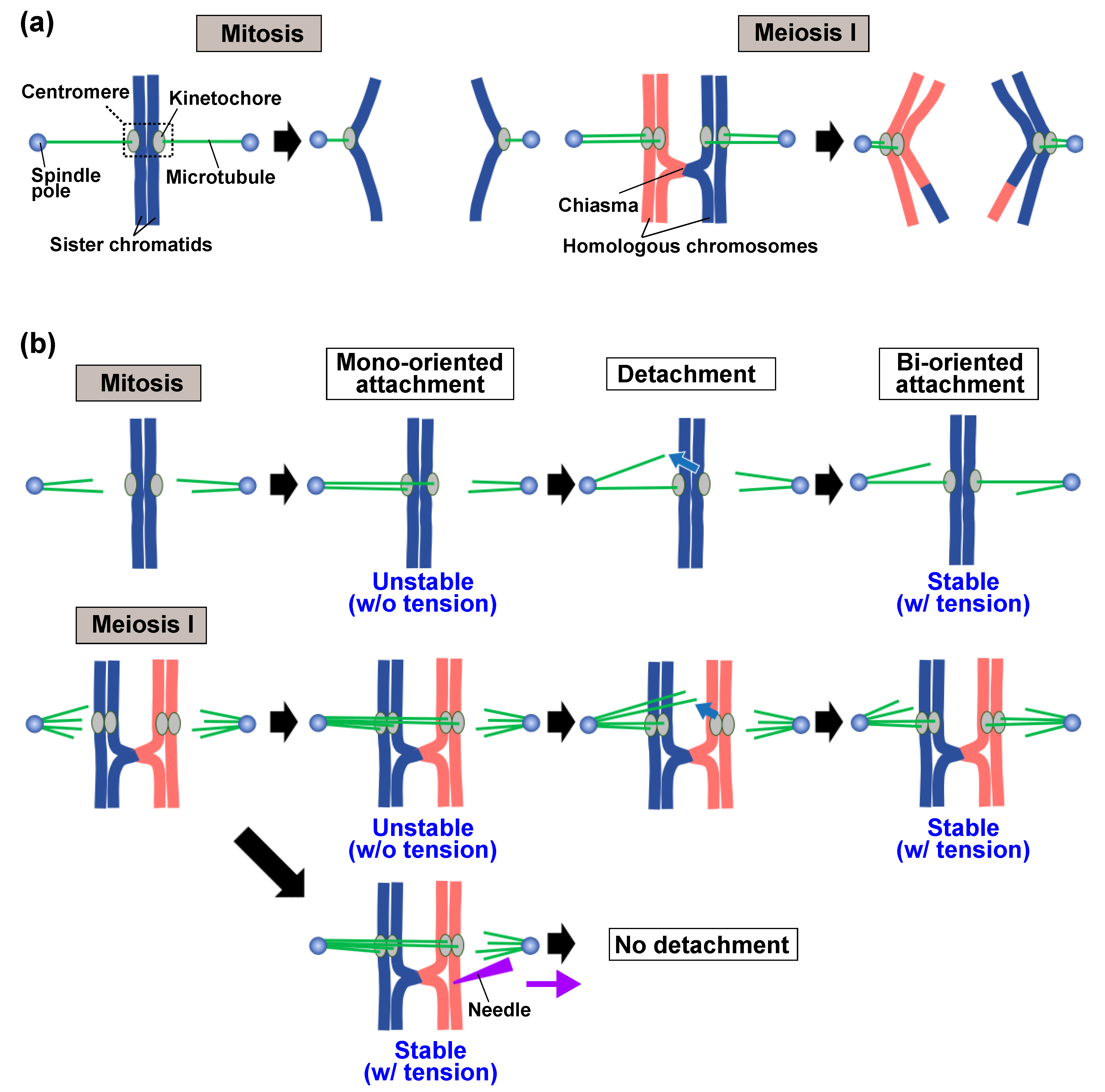This scientific diagram is divided into two sections, labeled A and B. Section A, located at the top, features two detailed diagrams—the left one illustrating the process of mitosis and labeled "mitosis" in black text within a grey rectangle, and the right one depicting meiosis I (denoted by a Roman numeral I in black text within another grey rectangle). Both diagrams use blue and red chromosome representations. Common elements in both diagrams are parts named centromere, spindle pole, sister chromatids, kinetochore, and microtubule. Additionally, the meiosis I diagram includes elements labeled chiasma and homologous chromosomes, illustrating more complex interactions between chromosome pairs.

Below this, Section B comprises three rows and further explores mitosis and meiosis I. In the top row, the progression of mitosis is shown through diagrams labeled as mono-oriented attachment, unstable without tension, detachment, and finally, bio-oriented attachment, which describe the stages in chromosomal alignment and separation. The second and third rows detail meiosis I. The second row addresses potential errors, depicting phases sequentially as meiosis I, unlabeled phase, unstable without tension, and stable with no tension. The third row clarifies the stable with tension condition in meiosis I. Green spindle fibers or "spindly things" highlight how they differently attach during these cellular processes. This diagram is color-coded, with blue and orange figures thought to represent chromosomes, providing a visual comparison of mitosis and meiosis I and their respective mechanics.